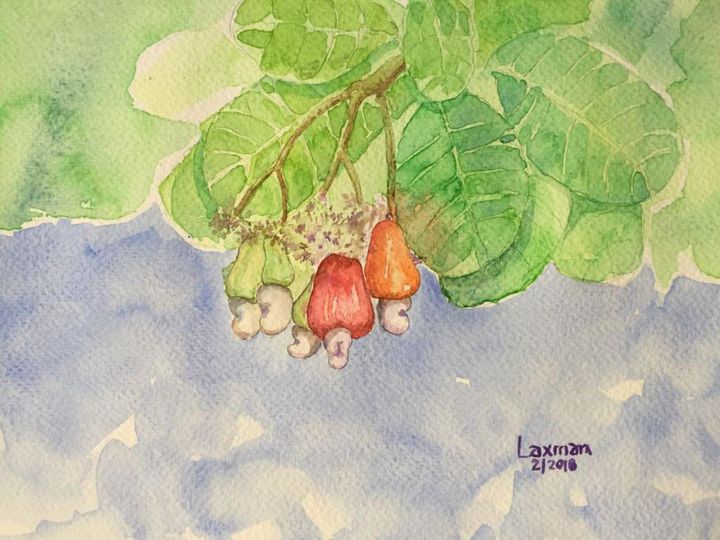This artwork appears to be an early attempt at a child-like drawing in a watercolor style. The image features a tree branch adorned with various fruits and mushrooms, vividly detailed with five distinct styles. Two mushrooms have yellow and green caps, while a smaller one is purely yellow. The branch also bears hanging fruit that resembles red and orange peppers, capped with white, lima bean-shaped tips. The scene is set against a blue, hazy sky that gives the impression it might be a reflection of water. Encircling this motif are large, rounded green leaves and clouds that serve as a container for the scene. The bottom right of the image has a watermark bearing the text "Laxman 2, 2018," marking its creator and year of creation.